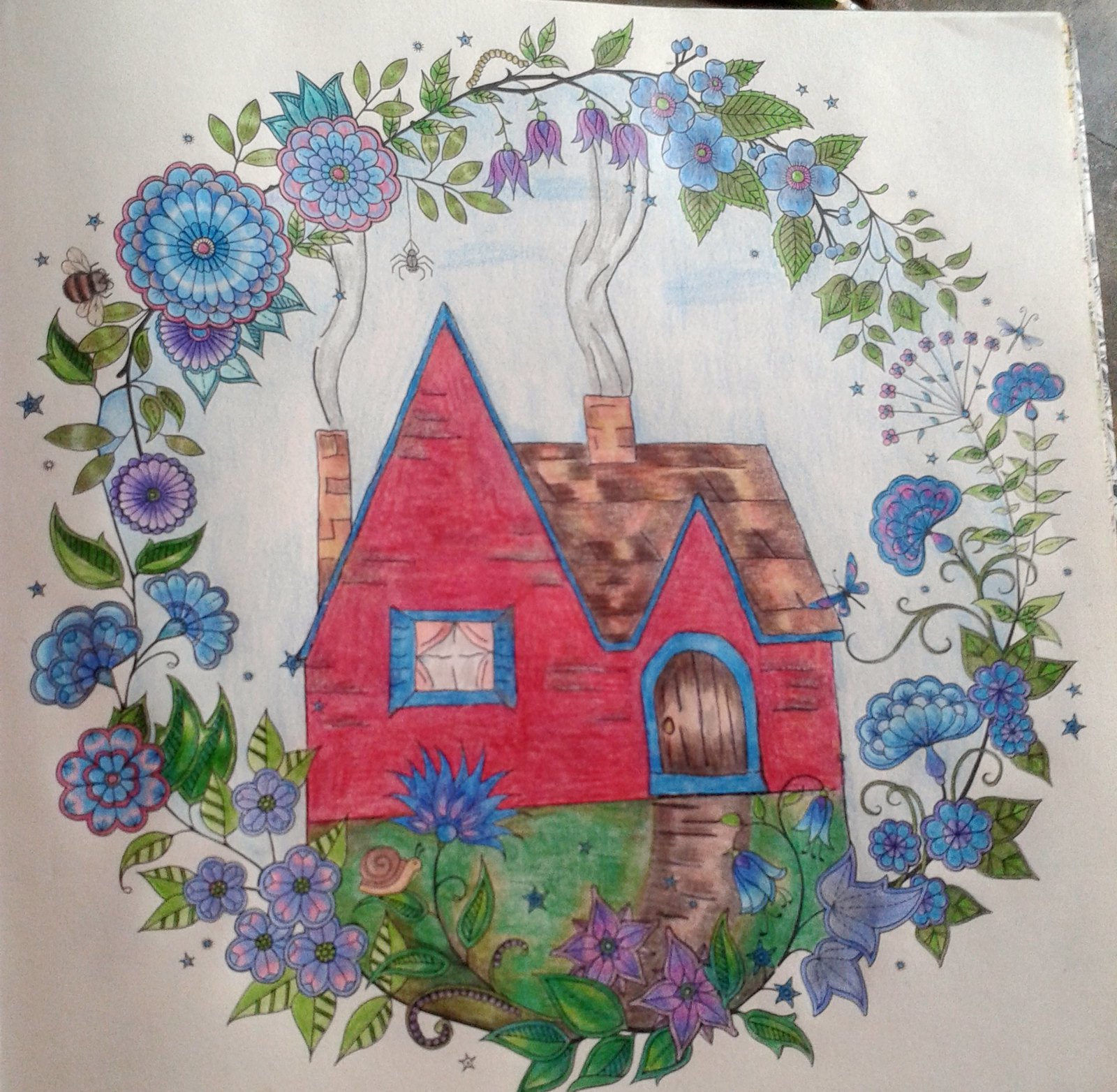The image is an intricately detailed drawing, executed with colored pencils on a piece of white paper. Dominating the scene is a quaint little house featuring a dual-peaked roof. The roof itself is rendered in shades of brown, complemented by two chimneys, also brown, each emitting a soft plume of smoke. The house is painted a vibrant red, adding warmth and charm to the composition. 

A single window, adorned with blue shutters and possibly pink curtains, provides a peek into the cozy interior. Below the window sits a brown door characterized by a straight bottom and an upper arch, framed by blue trim that accentuates its entryway. Leading up to the door is a dirt-colored path that meanders through the lush green grass of the front yard.

Encircling the entire scene is an array of flowers drawn on winding vines and stems, featuring green leaves interspersed with blossoms in shades of purple, blue, and various other colors. Amidst this floral border, a brown snail makes an appearance, adding a whimsical touch, although its exact position—whether on the yard or perched on a leafy plant—remains ambiguous. This detailed and colorful artwork captures a serene, storybook-like quality.